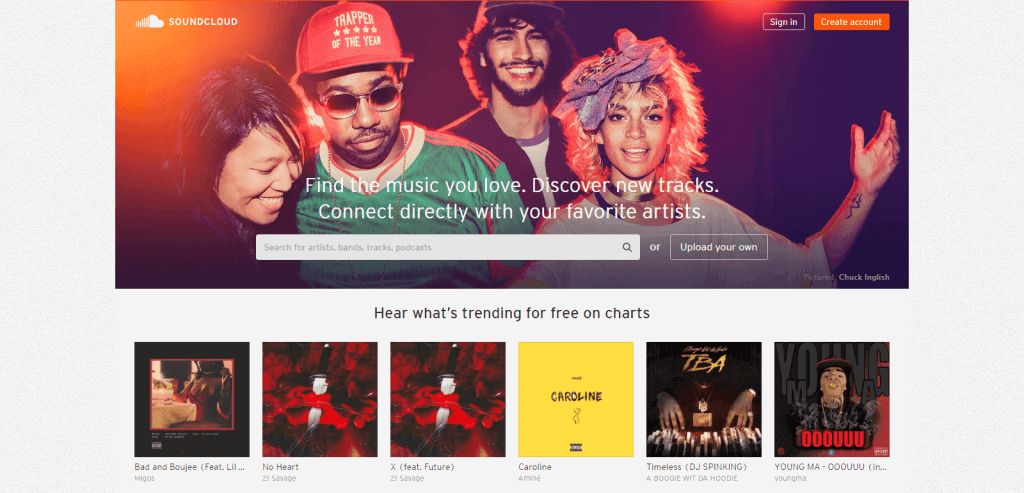This screenshot from the SoundCloud website features several elements that give a vibrant and inviting first impression. In the upper left corner, there is the iconic SoundCloud logo, which comprises a white cloud with three vertical bars cutting through its left side, accompanied by the capitalized 'SoundCloud' text to its right. In the upper right-hand corner of the interface, users can find the 'Sign In' button, and next to it, a prominent solid orange button labeled 'Create Account.'

The hero image dominating the center of the screen includes four individuals captured at night, bathed in an orangey glow. On the left, an Asian woman smiles warmly, surrounded by orange light leaks from the left and upper right of the scene. Next to her stands an African-American man sporting a vibrant red cap with the words "Trapper of the Year," sunglasses, and a likely green soccer jersey. Behind him, a Hispanic man is visible, also wearing a baseball cap. He exudes happiness with a smiling face, complete with a full beard, mustache, and shaggy hair. To his right, a young, light-skinned African-American woman appears. She has striking, potentially bleached or brightly-lit orange hair adorned with a large, purple, floppy bow. Her left arm is raised, revealing the palm of her hand and a tattoo on her wrist. She wears an oversized T-shirt along with noticeable metallic necklaces.

Overlaying this image is text inviting users to "Find the music you love, discover new tracks, connect directly with your favorite artists." A search field follows, accompanied by an additional option to "Upload your own." Below her, text states, "Here's what's trending for free on charts," showcasing six tracks: 

1. "Bad & Bougie" with its album cover.
2. "No Heart" and "X" featuring Future, both featuring the same logo of a knife through a heart on a yellow background with black text. 
3. "Caroline," though the album text appears slightly unclear.
4. DJ SpinKing's track, with some text mentioning "TBA" on the album cover.
5. Young M.A.'s "OOOUUU," featuring red text overlaying an image of the artist's face.

This detailed composition not only highlights SoundCloud's interface design but also emphasizes the platform's expansive and diverse musical offerings.